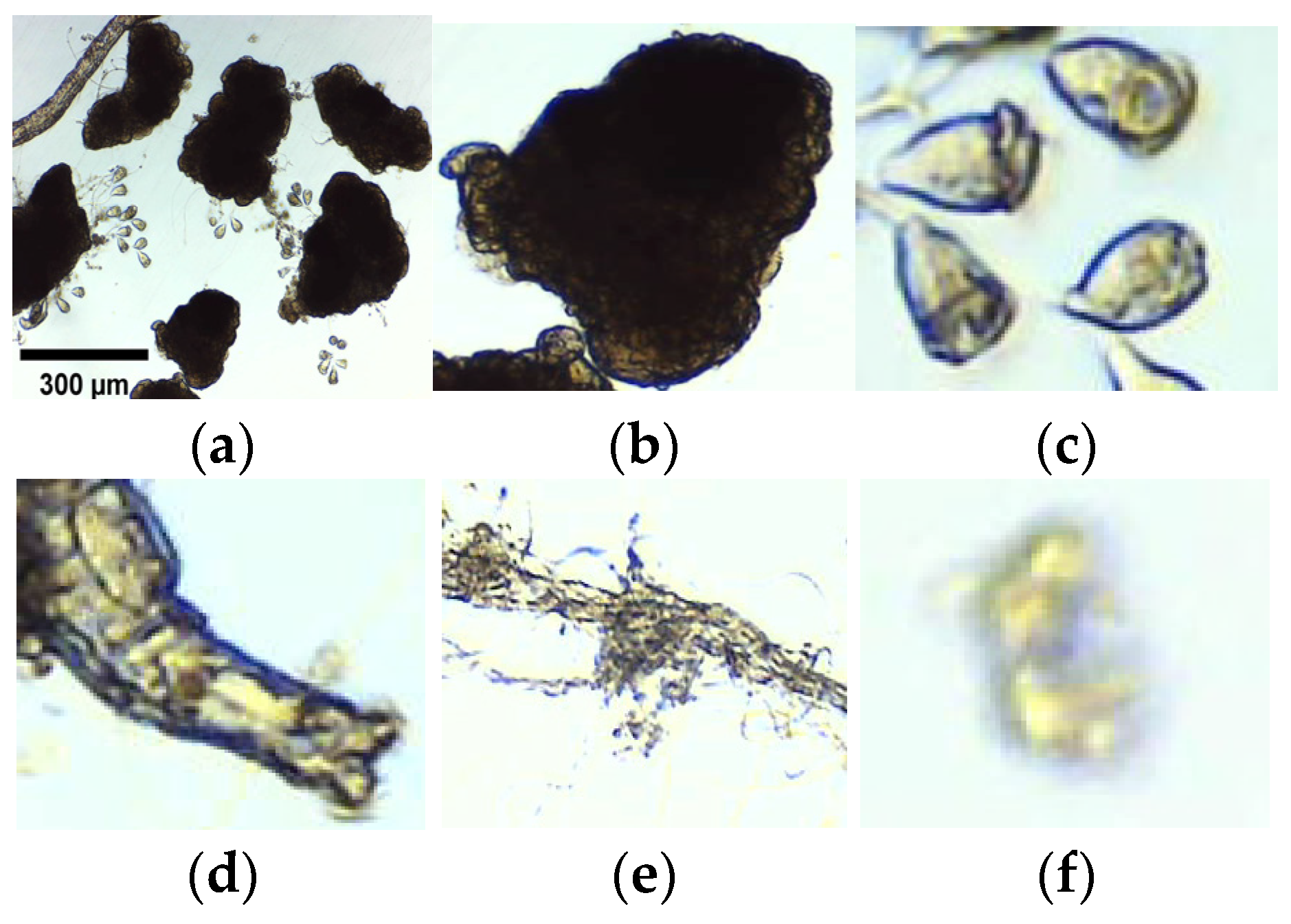This image consists of six equal squares displaying microscopic views, labeled A through F. Each square depicts different cells or microscopic organisms at 300 micrometers in scale. 

- **Square A:** Displays a dark field with multiple black blotches, potentially indicating densely packed cells or objects.
- **Square B:** Shows a large, dark black blob, possibly representing a large amoeba or similar organism.
- **Square C:** Contains several iridescent, clear-looking cells, about four to five in number, exhibiting intricate, translucent structures.
- **Square D:** Features a translucent cell with different colors diffused through it, resembling an elephant trunk in shape.
- **Square E:** Displays a cluster of dots, likely representing grouped cells or pollen particles.
- **Square F:** Contains a blurry image of a single organism or cell, with indistinguishable features but predominantly yellow.

This detailed microscopic series provides a diverse look at different microscopic entities, ranging from well-defined cellular structures to indistinct blobs.